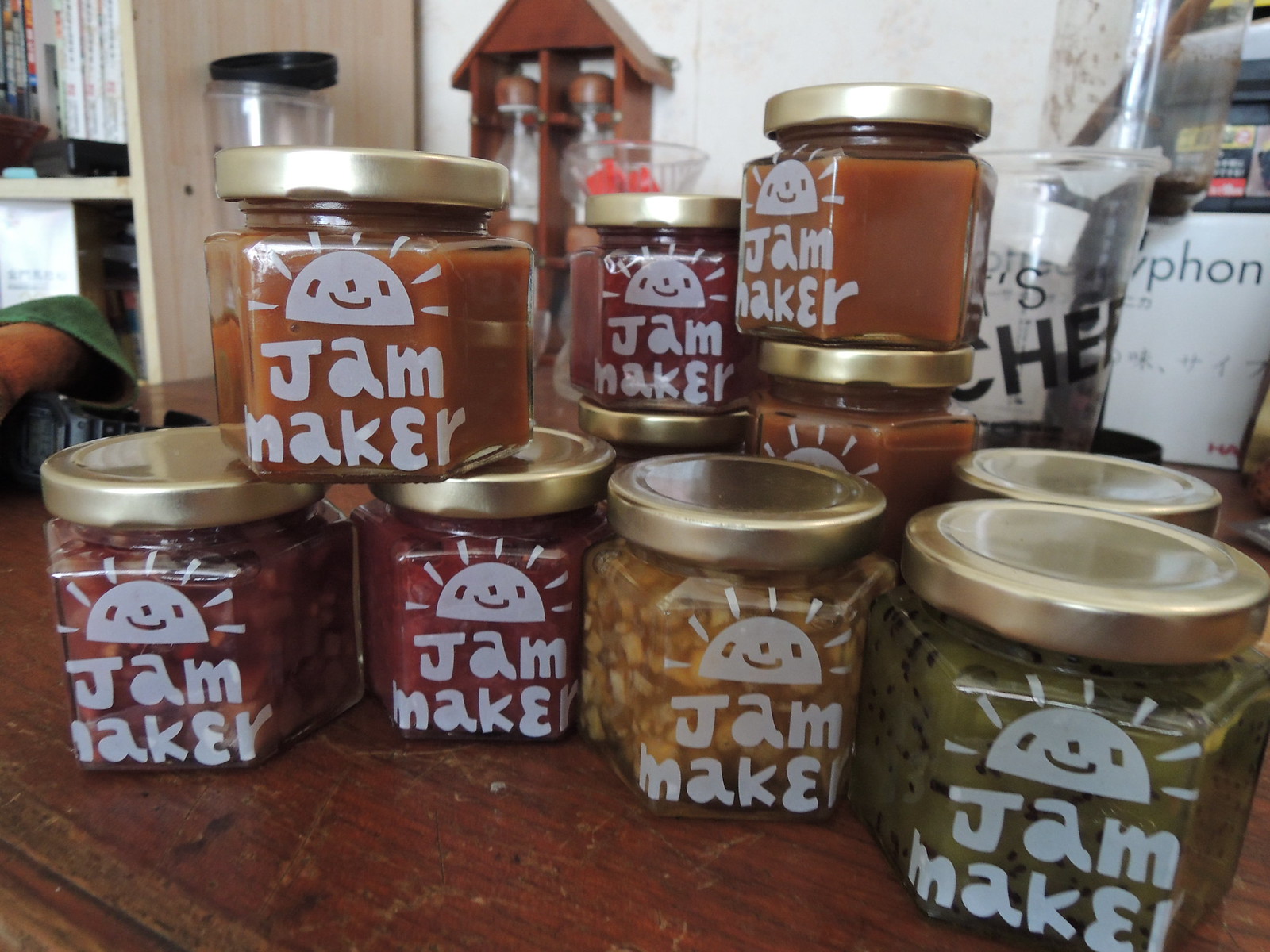This photograph captures a collection of ten identical six-sided, clear glass jars with plain metallic twist-on lids. Each jar features a stylized, smiling half-sun with square eyes and a cheery expression printed on the front, followed by the words "jam maker" in white letters. These jars are meticulously arranged on a heavily scratched and worn wooden table. The contents within the jars vary in color and texture: two contain a smooth, caramel-colored substance, two hold red preserves, one has a yellowy-orange substance resembling fruit marmalade, and one jar contains a green substance with dark flecks, possibly kiwi. Despite some clutter visible in the background, the focus remains on the orderly display of diverse jams, stacked thoughtfully to showcase the variety.